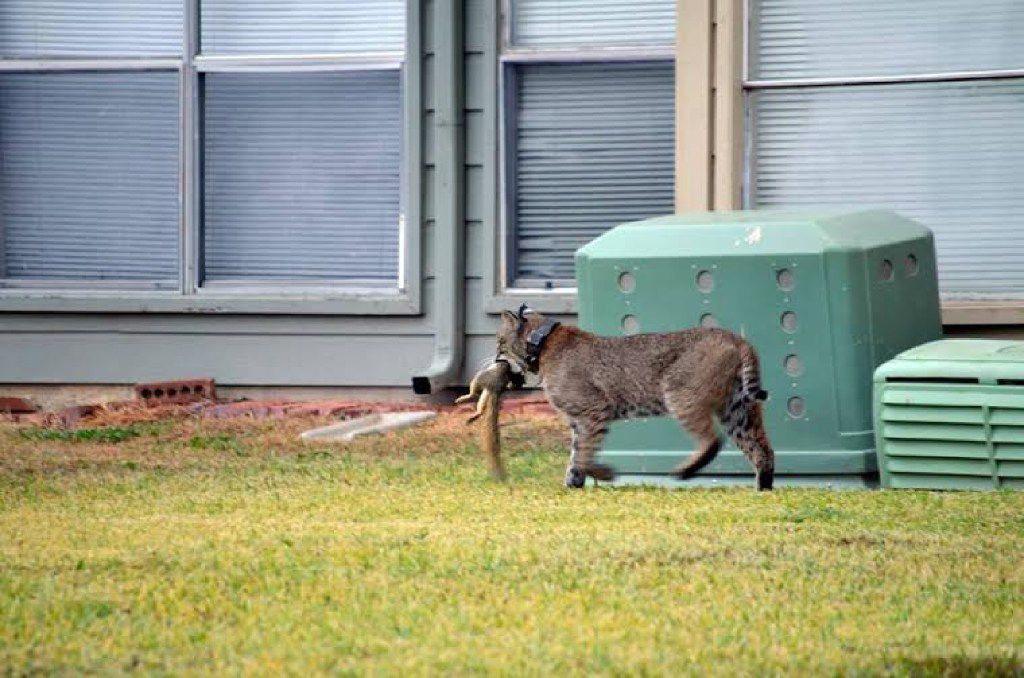In this slightly blurry color photograph, a robust bobcat, distinguished by a thick leather tracking collar around its neck, is captured mid-stride with a squirrel clutched firmly in its mouth, the squirrel's lifeless rear and tail visible. The scene unfolds in what appears to be a somewhat untidy backyard or possibly behind a business or factory, characterized by an eclectic mix of elements. The backdrop reveals large windows with various states of blinds – some fully drawn, others in disrepair. Air conditioning units or teal-green electrical boxes are positioned near the building, contrasting against the patchy green grass and red dirt ground. The bobcat's poised stance, with both its left front and rear paws lifted, underscores its stealth and agility as it moves from the right to the left of the photograph. The area also features utility elements such as a gutter system and dispersal bricks, emphasizing its functional rather than aesthetic purpose.